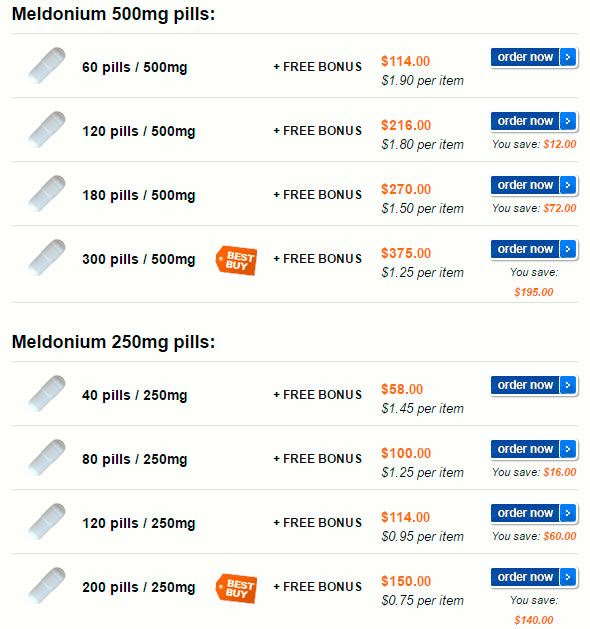The image displays a detailed breakdown of Meldonium pill pricing and quantities, categorized into two sections for 500mg and 250mg dosages. 

**Top Section: Meldonium 500mg Pills**
- The header shows "Meldonium 500mg Pills" in bold black text. Below, four rows each feature an image of a white pill capsule angled upwards and to the right.
  1. **60 Pills:** 500mg, including a free bonus. Priced at $114, which is $1.90 per pill. Includes a blue "Order Now" button with an arrow.
  2. **120 Pills:** 500mg, including a free bonus. Priced at $216, which is $1.80 per pill, offering a savings of $12. Features a "Order Now" button.
  3. **180 Pills:** 500mg, including a free bonus. Priced at $270, which is $1.50 per pill, saving $72. Comes with a "Order Now" button.
  4. **300 Pills:** 500mg, labeled as "Best Buy" on an orange tag, with a free bonus. Priced at $375, equating to $1.25 per pill. Provides a savings of $195 and includes an "Order Now" button.

**Bottom Section: Meldonium 250mg Pills**
- The header reads "Meldonium 250mg Pills," followed by four rows, each depicting a white pill capsule.
  1. **40 Pills:** 250mg, with a free bonus. Priced at $58, which is $1.45 per pill. Contains an "Order Now" button.
  2. **80 Pills:** 250mg, with a free bonus. Priced at $100, costing $1.25 per pill, saving $16. Includes an "Order Now" button.
  3. **120 Pills:** 250mg, with a free bonus. Priced at $114, making it $0.95 per pill, saving $60. Features an "Order Now" button.
  4. **200 Pills:** 250mg, labeled "Best Buy" on an orange tag, with a free bonus. Priced at $150, costing $0.75 per pill, providing a savings of $140. Includes an "Order Now" button.

Each "Order Now" button is highlighted, facilitating easy navigation to make a purchase. The detailed layout effectively outlines the diverse options available for potential buyers, emphasizing cost-efficiency and bulk-saving benefits.